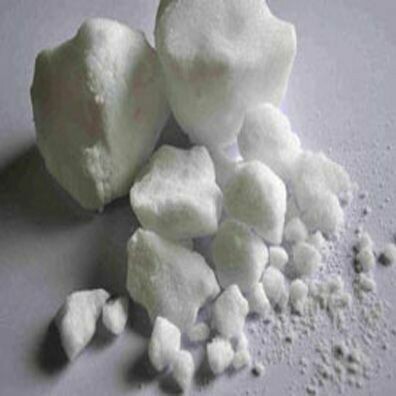The image is a square close-up featuring a gray background with various sizes of a white, crumbly substance distributed across it. Dominating the top left and top center are two irregularly shaped, somewhat rounded large chunks. In the middle, a smaller piece that resembles cottage cheese is noticeable, accompanied by a couple of similarly sized fragments to its right. As you move downward, the pieces progressively get smaller, finally transitioning into a fine powder at the bottom right corner. The lighting from the top right casts noticeable shadows to the bottom left of the larger chunks, highlighting their texture and irregular shapes. The image has no writing or text, depicting a gradient from larger white blocks at the top left to tiny crumbs and powder at the bottom right. The scene could be of sugar, salt, or a fragile rock-like substance, possibly set in a kitchen or an outdoor environment.